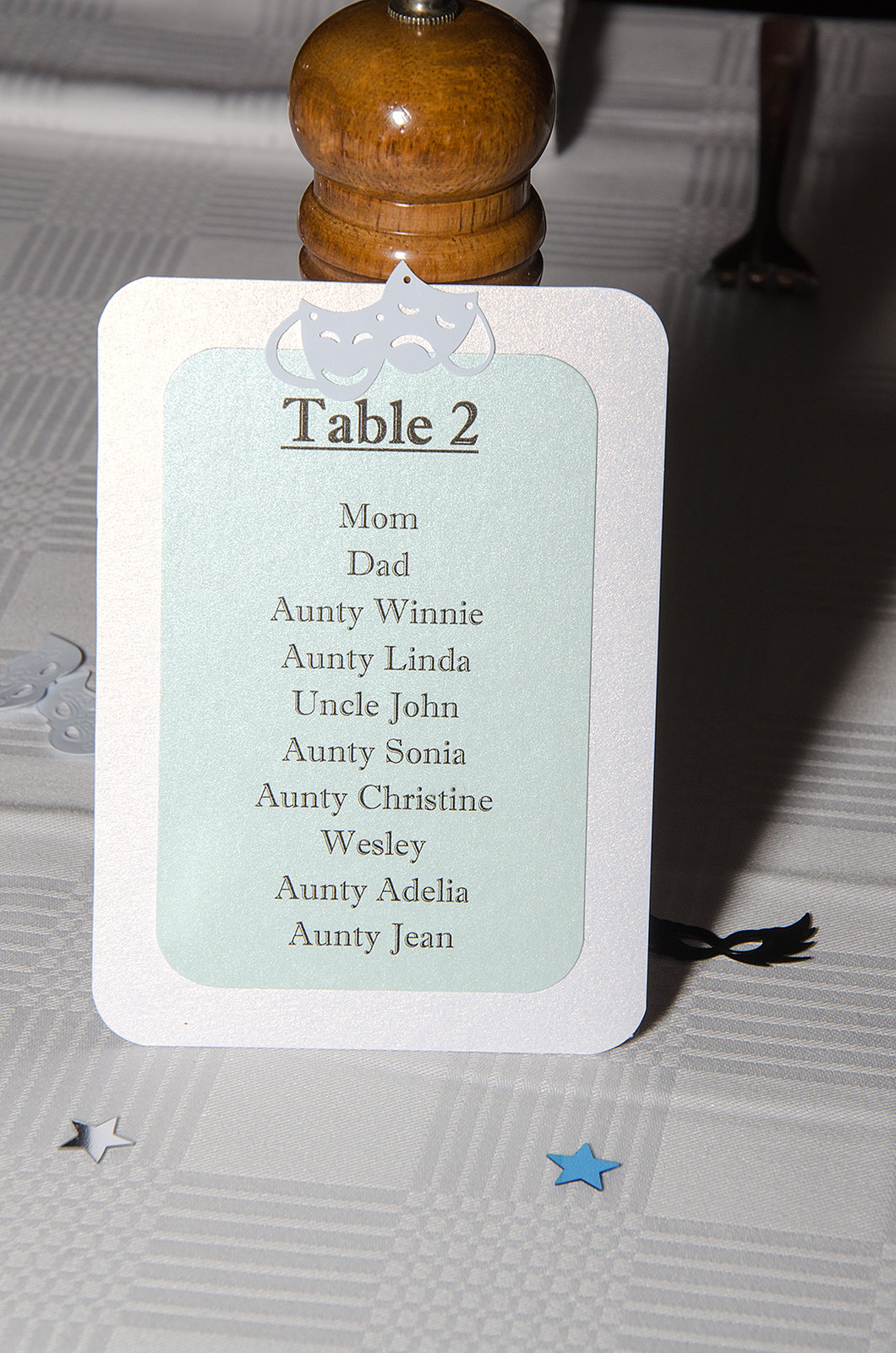This image captures a detailed table arrangement, prominently featuring a wooden pepper grinder that supports a folded card. The table is draped with a white cloth adorned with a pattern of intersecting squares. Scattered across the table are metallic stars in blue, silver, and possibly other colors, adding a festive or celebratory touch. Around the pepper grinder, there's a small black mask and other theatrical masks depicting the themes of happiness and sadness, likely representing a dinner theater setting. The card itself appears to have a blue background mounted onto a white base, with black text listing names in a familial sequence: "Mom, Dad, Auntie Winnie, Auntie Linda, Uncle John, Auntie Sonia, Auntie Christine, Wesley, Auntie Adalia, and Auntie Jean." This is designated as "table two," suggesting it’s part of a larger organized event. A fork and knife subtly placed in the background, along with the decorative stars, enhance the table's elegance and thematic elements.